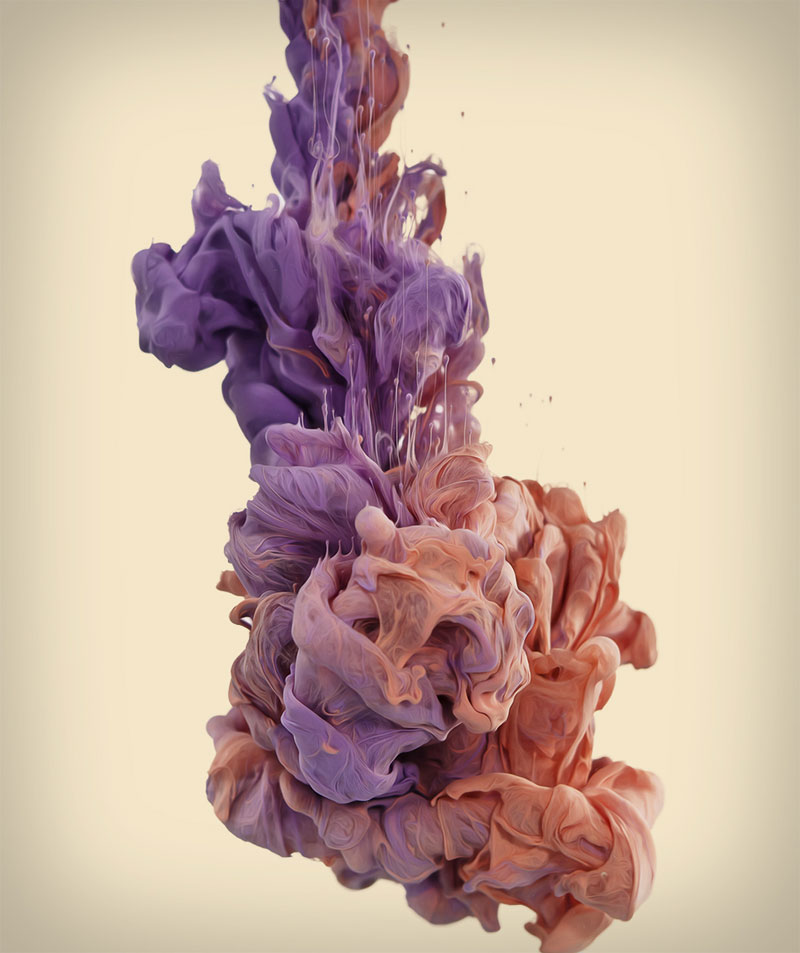The vertically rectangular image features an abstract scene with fluid transitions of neutral background colors, blending from grays at the corners to a nearly flush tone in the center. Dominating the foreground is a delicate form that evokes the imagery of cloth or dye diffusing in water. This central element starts with rich purples mixed with light brick red and gray hues at the top, gradually swirling and expanding into peachy pink and orangish tones toward the bottom. The object has an ethereal, almost floating quality, resembling either a ruffled, knotted scarf immersed in water or vibrant food coloring slowly dispersing through a liquid, creating a sense of movement and transformation within the stillness of the image.